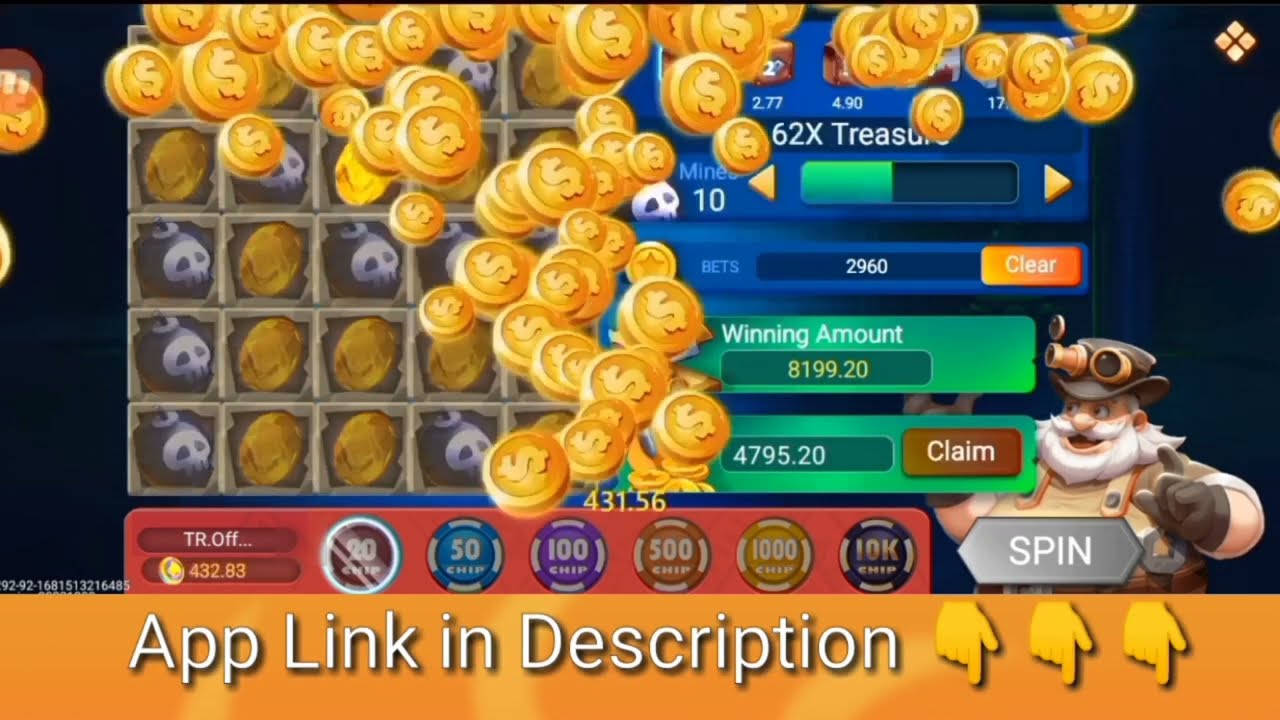In this image, we see an advertisement for a gambling video game. Dominating the scene are numerous gold coins cascading down like from a casino machine or treasure chest, creating an impression of abundance and excitement. At the top, the word "Treasure" is boldly displayed, and just below it, detailed numeric values are stated: a winning amount of 8199.20 and another figure of 4795.20, accompanied by a button labeled "Claim."

To the left, we see numerical indicators such as "bets 2960" and "62 X treasure." Nearby, several poker chip images are present, displaying values of 20, 50, 100, 500, 1000, and 10k. A man, depicted as a cartoon character, appears at the bottom left of the screen. He is somewhat overweight, with a gray beard and mustache, and white hair. His attire includes overalls, gloves, and a hat adorned with binocular-style lenses. The man is smiling, raising a finger as if addressing the viewer, and to his right, the word "Spin" stands prominently.

At the very bottom of the screen, a yellow banner stretches across, bearing the words "app link in description" and flanked by three images of fingers pointing downwards, urging the viewer to take action. The entire scene is vibrant with details and imagery designed to evoke the thrill of potential winnings and discovery.